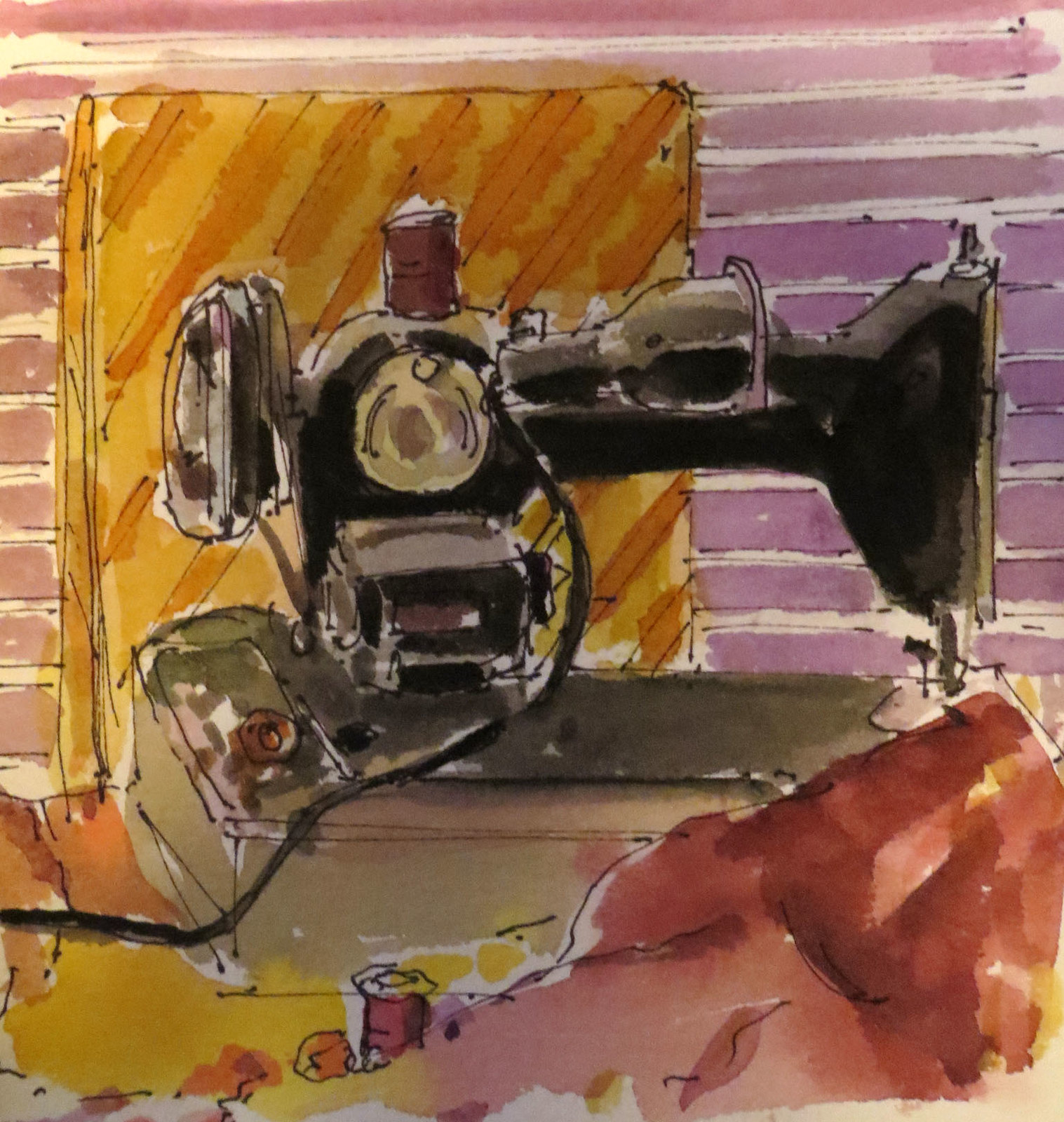This watercolor painting captures a vintage sewing machine reminiscent of the classic Singer models from over half a century ago. The machine, devoid of any fabric under its needle, takes center stage, with intricate details that highlight its nostalgic charm. Adjacent to the sewing machine lies a substantial piece of red fabric, accompanied by a spool of matching red thread, suggesting an imminent sewing project. An electrical cord extends from the machine, trailing off to the left, hinting at its power source. The backdrop features a wall adorned with purple stripes and a beige book positioned right behind the sewing machine. The painting is grounded by a beige floor, adding a subtle contrast to the vivid colors and intricate details of the sewing setup. This piece beautifully combines elements of nostalgia and artistry, evoking a sense of timeless creativity.